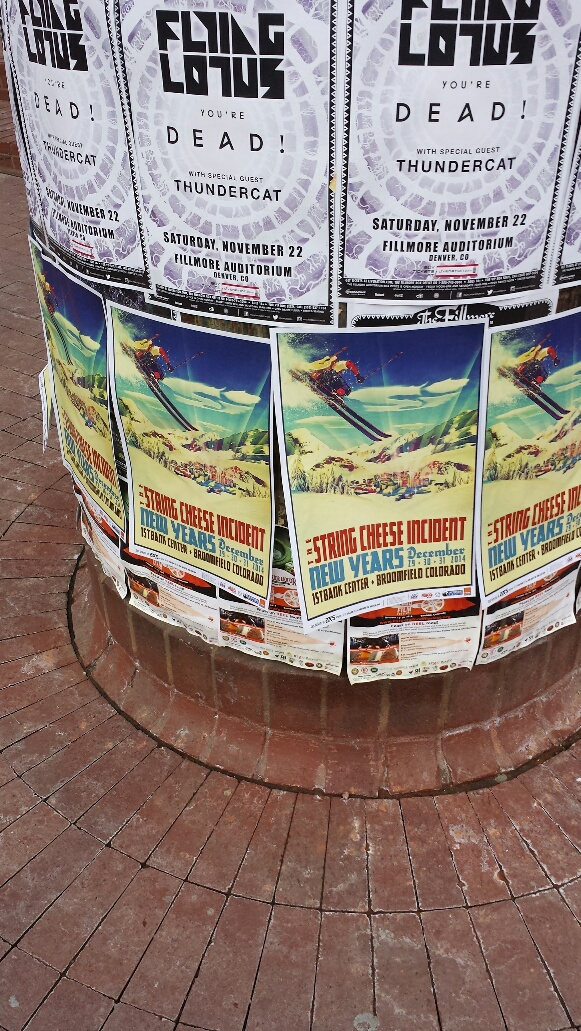The vertical rectangular image features a thick outdoor column or pillar, used for posting advertisements, standing on a tiled or brick floor that shares the same pattern as the pillar. The viewer's perspective is from someone standing in front of the pillar and looking down. Surrounding the base, there's a ring of identical white posters with black lettering, prominently advertising a Flying Lotus concert with the text, "Flying Lotus, You're Dead with special guest Thundercat, Saturday, November 22nd, Fillmore Auditorium, Denver, Colorado." Above this, another ring of posters displays a mountain and lake scene with an image of a skier, promoting The String Cheese Incident's New Year's event at the First Bank Center in Broomfield, Colorado, set for December 2014. The entire column is densely covered with these overlapping posters, highlighting the vibrant promotional material in an outdoor setting.